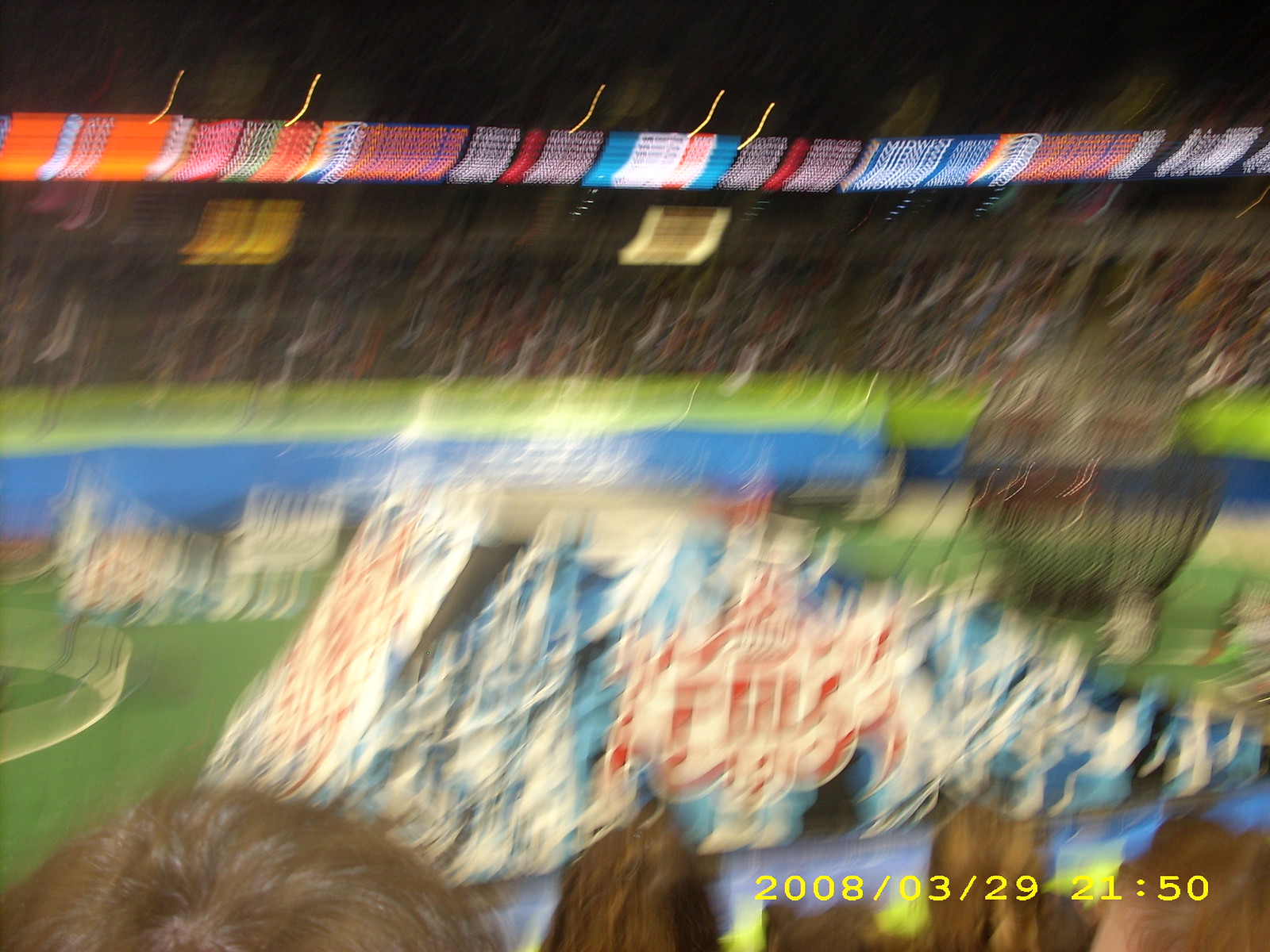This photograph, taken inside a bustling arena, captures a moment frozen in time on March 29, 2008, at 21:50, as indicated by the timestamp in the bottom right corner. Despite its blurriness, the image reveals key details: in the center of the field, a large, mysterious object covered by a blue and white striped tarp with a symbol featuring red writing and a red outline is prominently displayed. The bright stadium lights encircle the arena, delineating the separation between the lower and upper levels of the crowded bleachers, which are filled with spectators. Directly below the bleachers is a distinct green strip followed by a blue strip, leading to the expansive green field at the bottom of the image.